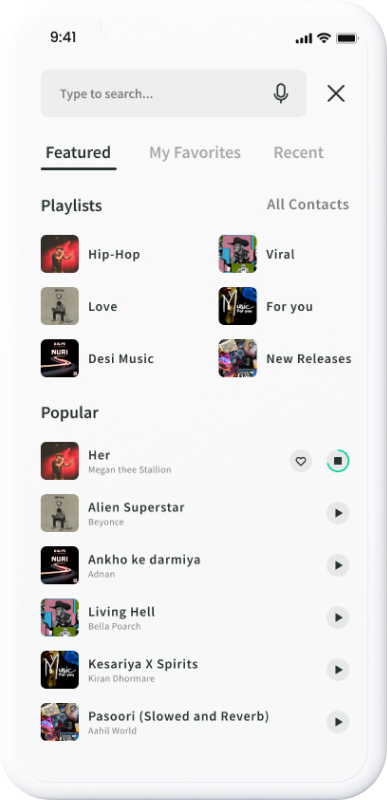This image features a detailed view of a mobile music application displayed on a white smartphone. The phone itself serves as the frame, with the screen featuring a predominantly white background. 

At the top of the display, the status bar is visible. The left corner shows the time as 9:41, while the right corner features icons indicating strong cell signal, Wi-Fi connectivity, and a nearly full battery at approximately 97-98% charge.

Just below the status bar, there is a search bar labeled "Type to search," which includes a microphone icon allowing voice search functionality. To the right of the search bar, a black 'X' icon is available to clear the entered text or close the search.

Further down, there are three black tabs: "Featured," "My Favorites," and "Recent," with a black underline beneath "Featured," indicating the active section. Below these tabs, options for "Playlist" and "All Contacts" are present.

Further down the screen, the "Popular" section showcases a list of trending songs by notable artists such as Megan Thee Stallion ("Her"), Beyoncé, Adnan, Bella Poarch, Kieran Daufmeyer, and Aaliyah Whirl. One of the songs is marked with a heart icon, signifying it as a favorite, and the currently playing song is indicated by an active play bar. The progress of the song is visually depicted by a green-outlined stop button, showing how much time is remaining.